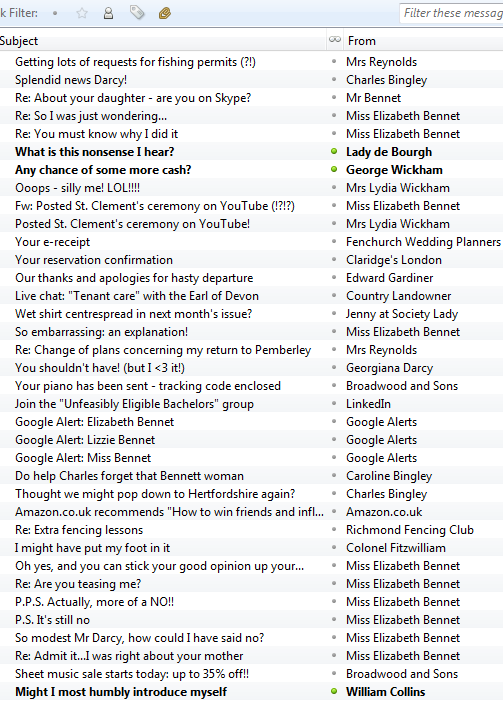The image displays a user interface, likely an email or messaging application, featuring a cluttered inbox with numerous messages. At the top, there's an action bar with icons including a filter, a star, a profile, a price tag, and a paperclip, suggesting functionalities like marking important messages, viewing profiles, or attaching files. Beneath this bar, a filter option allows users to sift through messages, perhaps to manage the high volume of approximately 35-40 options listed vertically.

Each message preview includes a subject and sender. Notable entries include:
- "Getting lots of requests for fishing permits?" from Ms. Reynolds.
- "Splendid news, Darcy," from Charles Bingley.
- "Ari, about your daughter, are you on Skype?" from Mr. Bennett.
- "Re: So I was just wondering," from Ms. Elizabeth Bennett.
- "Re: So you must know why I did it," from Ms. Elizabeth Bennett.

Highlighted messages, indicated by bold text and large green dots next to the names, imply unread or important communications:
- "What is this nonsense I hear?" from Lady Deboro.
- "Any chance of some more cash?" from George Wickham.
- "Might I most humbly introduce myself," from William Collins.

The remaining messages display with gray dots, indicating lower priority or read status. The overall scene suggests a context rich with character interactions, potentially part of a narrative, story-driven game, or interactive puzzle, given the mixture of familiar names and dramatic subject lines.